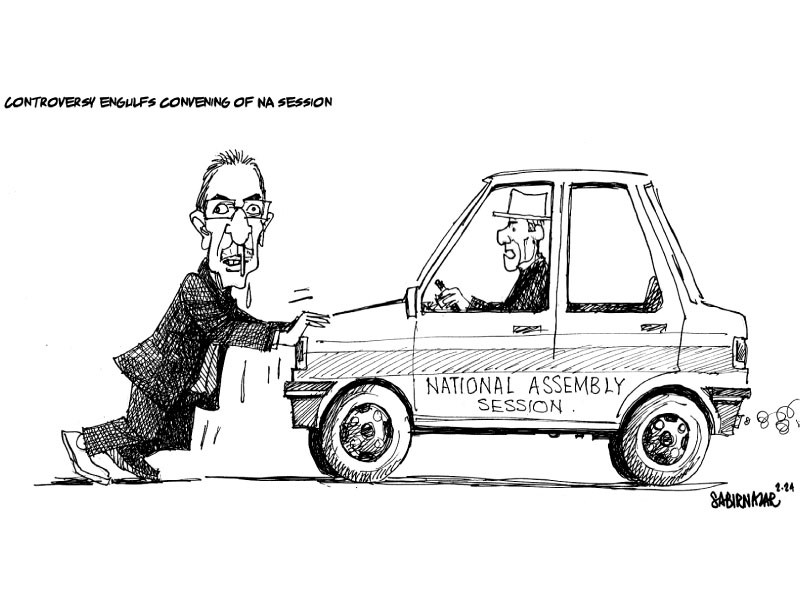In this black and white hand-drawn comic panel, a man in a baggy suit, with comically exaggerated features including a large nose, chin, and ears, is depicted struggling to push a small car labeled "National Assembly Session." The man pushing the car is visibly straining, with sweat and possibly drool dripping from his face, while he stares directly at the viewer through glasses. The car appears to be driven by another man who is grimacing and gripping the steering wheel angrily. Exhaust is billowing from the car’s rear, enhancing the sense of effort and strain. Above the illustration, text reads "Controversy Engulfs Convening of N.A. Session," underscoring the chaotic scene. The artist's signature is visible in the lower right-hand corner, emphasizing its authenticity.